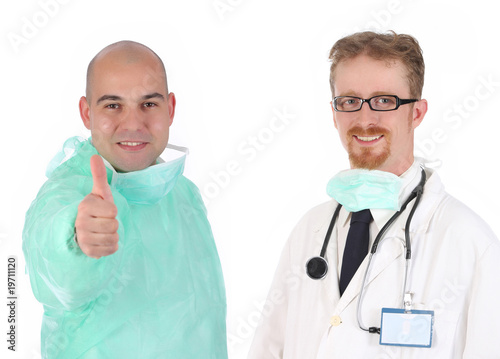This image features two male doctors standing side-by-side against a white background with "Adobe Stock" written repeatedly in gray block letters. The doctor on the left is bald, has brown eyebrows, and is dressed in light green scrubs. He is smiling slightly with his mouth open, showing a bit of his teeth, and is giving a thumbs-up with his right hand. The doctor on the right has ginger hair, a goatee, and is wearing black-framed glasses. He is dressed in a white lab coat with a beige button, a black tie, and has a stethoscope around his neck. A blue hospital mask hangs around his chin, and he has a blue-and-white name tag clipped to his coat. A vertical line with the number 1971120 and "Adobe Stock" is visible on the lower left part of the image.